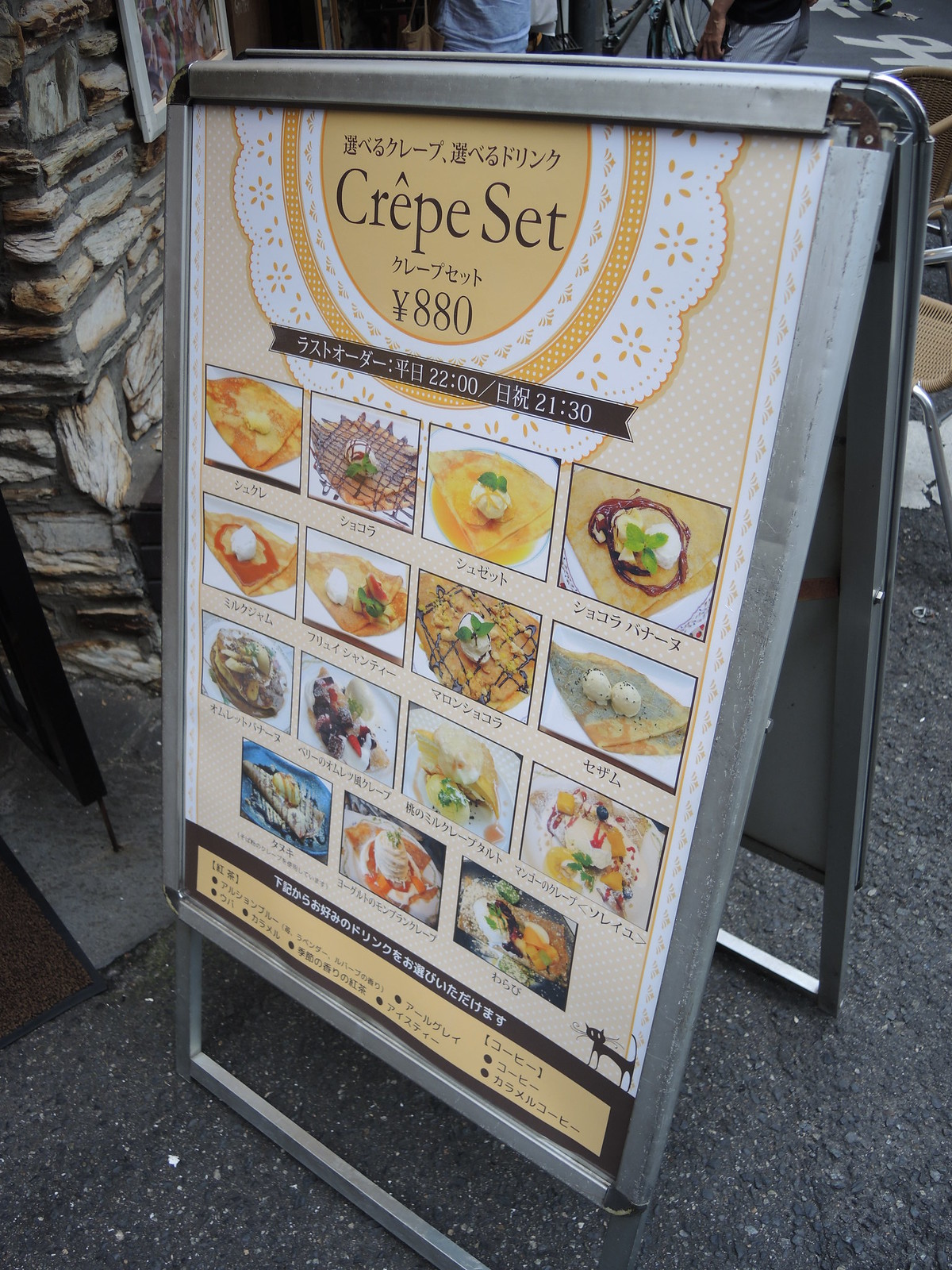The image depicts a folding metal menu board, likely situated outside a Japanese restaurant, as suggested by the presence of Japanese writing and the mention of prices in yen. The board displays the word "Crepe Set" prominently in English, with other text in Japanese, and lists a price of 880 yen. It is designed like a letter V when unfolded, standing on what appears to be blacktop or a sidewalk, and positioned near a stone wall with possible pedestrian activity seen in the background.

The board features four rows of pictures showcasing various desserts, likely different kinds of crepes or waffles, each artistically decorated. The top three rows each contain four images of these desserts, while the bottom row has three images. These pictures are centered around the food items, which are elaborately adorned with various toppings such as chocolate and whipped cream. Additionally, there are operational times listed as 22:00 and 21:30, suggesting the restaurant's open hours on certain days.

In the bottom right corner of the menu, there is a small depiction of a black cat, adding a distinctive and charming touch to the board. This detailed and visually appealing board serves to inform and entice potential customers about the dessert offerings available inside the restaurant.